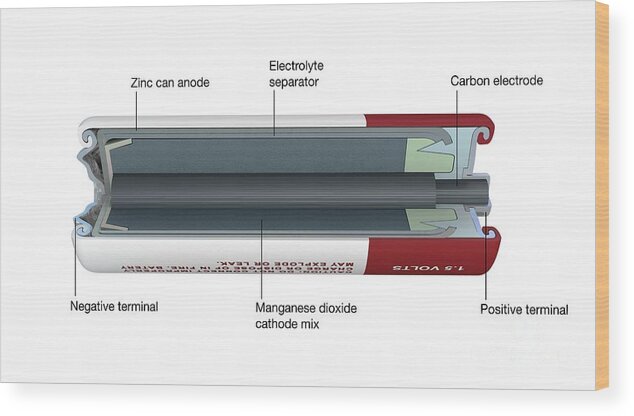This image is a detailed 3D canvas print of a cylindrical battery cut in half to reveal its internal components, set against a white background with tan sides featuring a wood grain overlay. The battery is displayed laying sideways, with its top, colored burgundy red, positioned to the right, and its bottom, colored white, to the left. The outer casing of the battery is gray, while the inside showcases shades of gray and a hint of green. 

The print details various labeled parts of the battery, including the Positive Terminal, Carbon Electrode, Electrolyte Separator, Manganese Dioxide Cathode Mix, Zinc Can Anode, and the Negative Terminal. The battery is specified as 1.5 volts, with the labeling on the battery appearing upside down. At the base of the battery, there is a warning text that reads "may explode or leak."